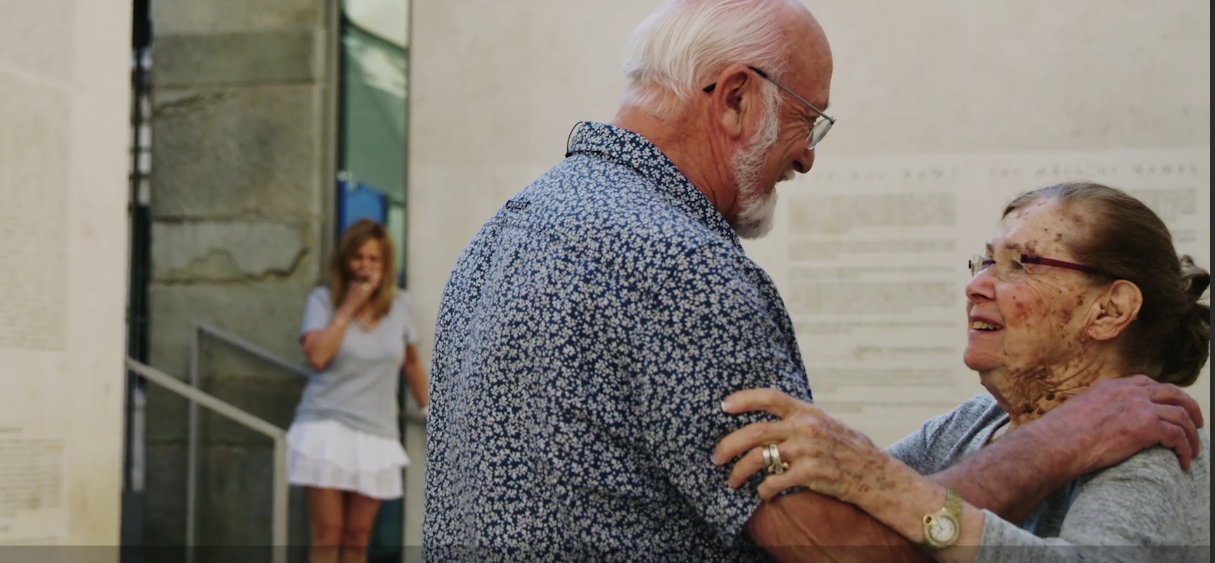The image captures a heartfelt moment between an elderly couple and a woman standing on a staircase in the background, surrounded by a cream-colored wall and a grayish-brown door or pillar. The elderly man, slightly tall with a receding hairline, gray hair, and a white beard, is wearing a navy short-sleeved shirt adorned with a white floral pattern and glasses. He tenderly embraces the elderly woman in front of him, placing a hand on her shoulder. The woman, shorter in stature with brown hair pulled back, is dressed in a gray sweater and also wears glasses. Her freckled face and hands, marred by some skin condition, do not dim her joy as she gazes up at the man, smiling warmly. Their embrace and mutual gaze of affection form the focal point of the image. In the background, standing on a staircase, is a younger woman in her late forties with shoulder-length brown hair. She is dressed in a gray top and a white miniskirt, anxiously holding her right hand to her mouth while observing the couple. The photograph, slightly blurry, is a vivid tableau of love and emotional connection.